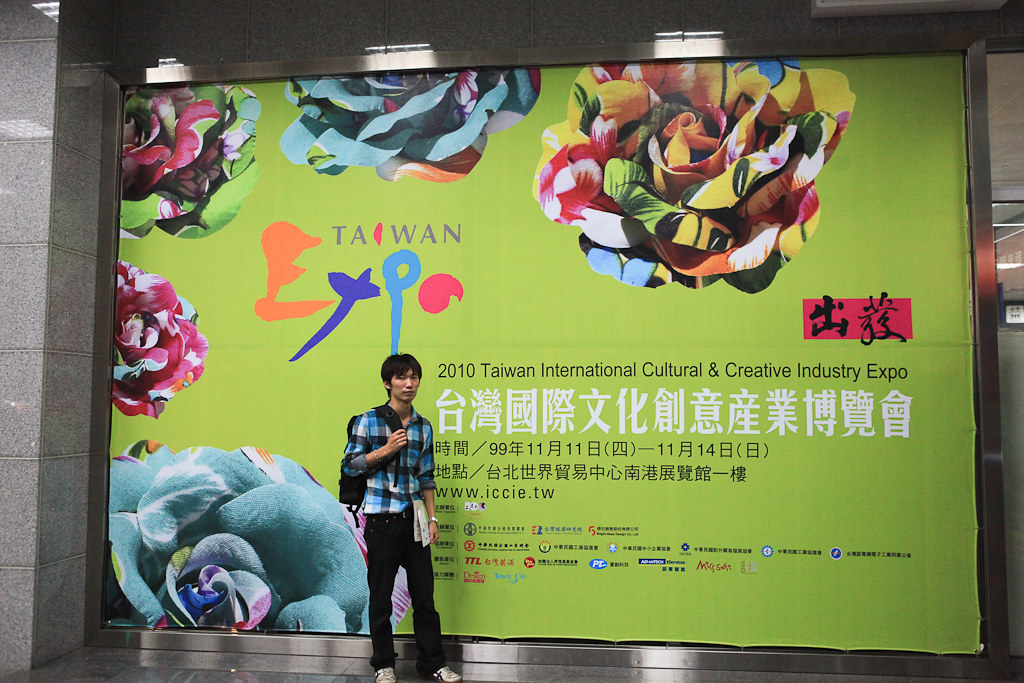A young man, likely in his late teens or early 20s, stands before a large, vibrant sign with a green background. The sign prominently reads "2010 Taiwan International Culture and Creative Industry Expo" with the words "Taiwan Expo" painted in various colors: 'E' in orange, 'X' in purple, 'P' in blue, and 'O' in dark pink. Surrounding the man, who wears a blue and black plaid shirt, dark jeans, and white and black tennis shoes, are multicolored flowers resembling roses in hues of blue, pink, white, yellow, orange, and green. He holds a bag behind him and papers in his left hand. The sign includes white Asian characters, logos of different countries or companies at the bottom, and the website www.iccie.tw.